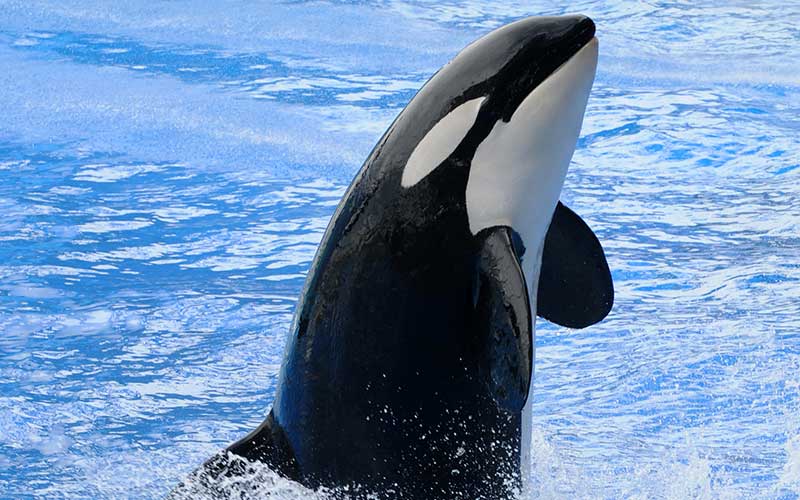The photograph captures a striking image of an orca, or killer whale, leaping almost vertically out of brilliant blue water. The orca is centrally positioned in the frame, with its sleek body extending from its nose to the top of its dorsal fin prominently visible. Its iconic black and white coloration is on full display: the white false eye spot, the white patch on its chin, and its black flippers and dorsal fin contrast sharply with the water. The texture of the water suggests it is within a tank, resembling the clear, uniform blue often seen in swimming pools, rather than the variable shades of the open sea. The orca's body shows no visible scars or imperfections, highlighting its pristine condition. As the orca arches slightly to the right, white froth is visible at the base, indicating the force of its powerful ascent. The water surface is relatively calm, adorned with subtle wave patterns and illuminated by gentle reflections of light.